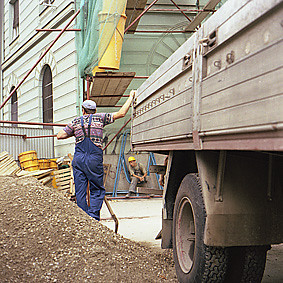The photograph showcases a detailed urban construction scene. Dominating the center is a man in blue overalls with blue suspenders, a multicolored short-sleeved t-shirt, and a gray cap, standing with his back to the camera. His right hand rest on the wooden side of a trailer, which has two large black wheels and mud flaps visible on the right side. To the left of the man is a pile of brown dirt or gravel, with several barrels and orange buckets nearby.

In the background, a tall building with contrasting façades—green on one side and beige on the other—features high arched windows on the beige side. Scaffolding is erected along the building, and two large yellow tubes used for debris removal extend downward. Below the scaffolding, another man wearing overalls and a yellow hardhat is seated.

The scene is rich with construction details, including a temporary fence lined with pallets, boxes, and crates, adding to the industrious atmosphere of the site.